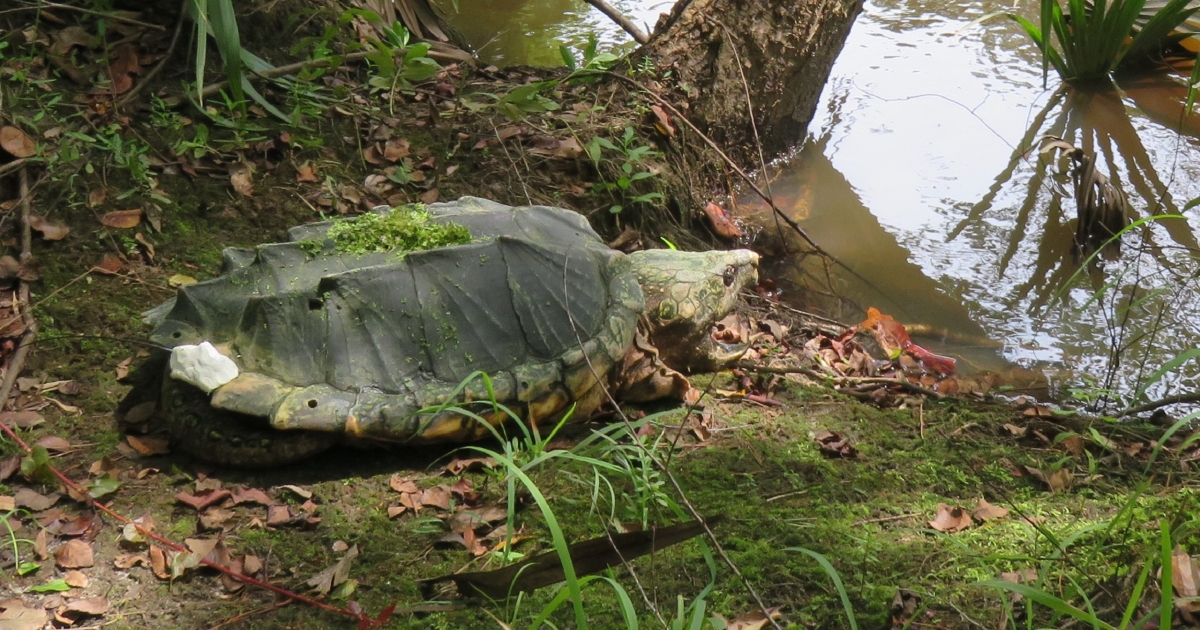In this outdoor photograph, we see a distinguishably old tortoise poised at the brink of a murky body of water—possibly a river, swamp, or stream—where it seems to be contemplating entering. The tortoise's shell is a striking feature, characterized by two distinct spiny ridges running lengthwise, each adorned with mildly pointed edges that make it stand out. The shell itself is predominantly black with patches of green moss and some scattered leaves, lending an earthy, ancient appearance. The tortoise, with its greenish head and partially visible eye, appears to be navigating through an environment rich in plant life, including moss, grass, and nearby trees leaning into the water. The water is notably dark and opaque, suggesting a muddy bottom typical of such ecosystems. Additionally, the underside of the tortoise carries a yellowish-green hue, further complementing its rugged, natural setting.